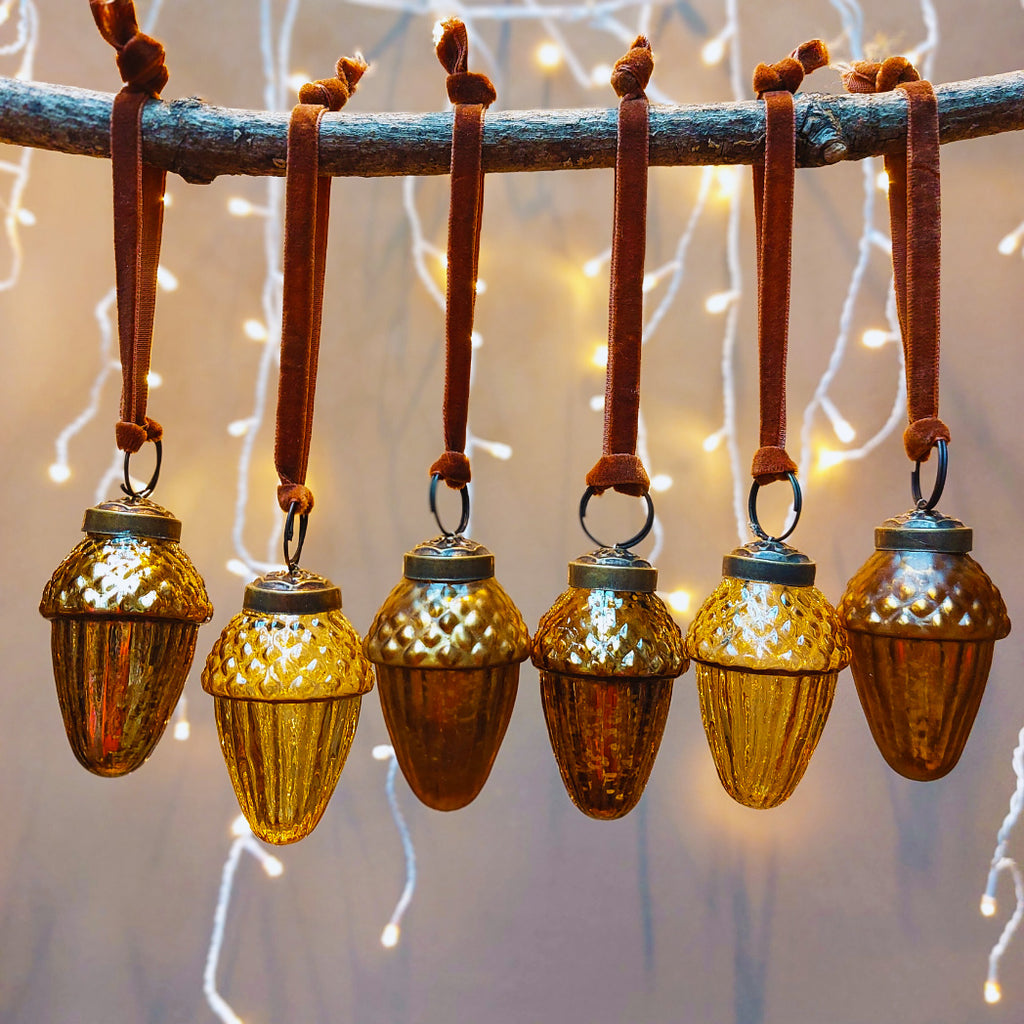This square photograph features a horizontal tree branch at the top, from which six acorn-shaped glass ornaments hang. The ornaments are attached to the branch with brown suede cords, knotted securely at the top. Each ornament has a textured silver cap, with the upper portion adorned with dots and the bottom showcasing vertical grooves leading to a rounded, narrow base. The colors of the ornaments vary: the one on the far left is brown, followed by a gold ornament, then two brown ones in the middle, another gold, and a final brown ornament on the far right. In the blurry background, white string lights dangle down, creating a festive, twinkling ambiance reminiscent of Christmas décor.